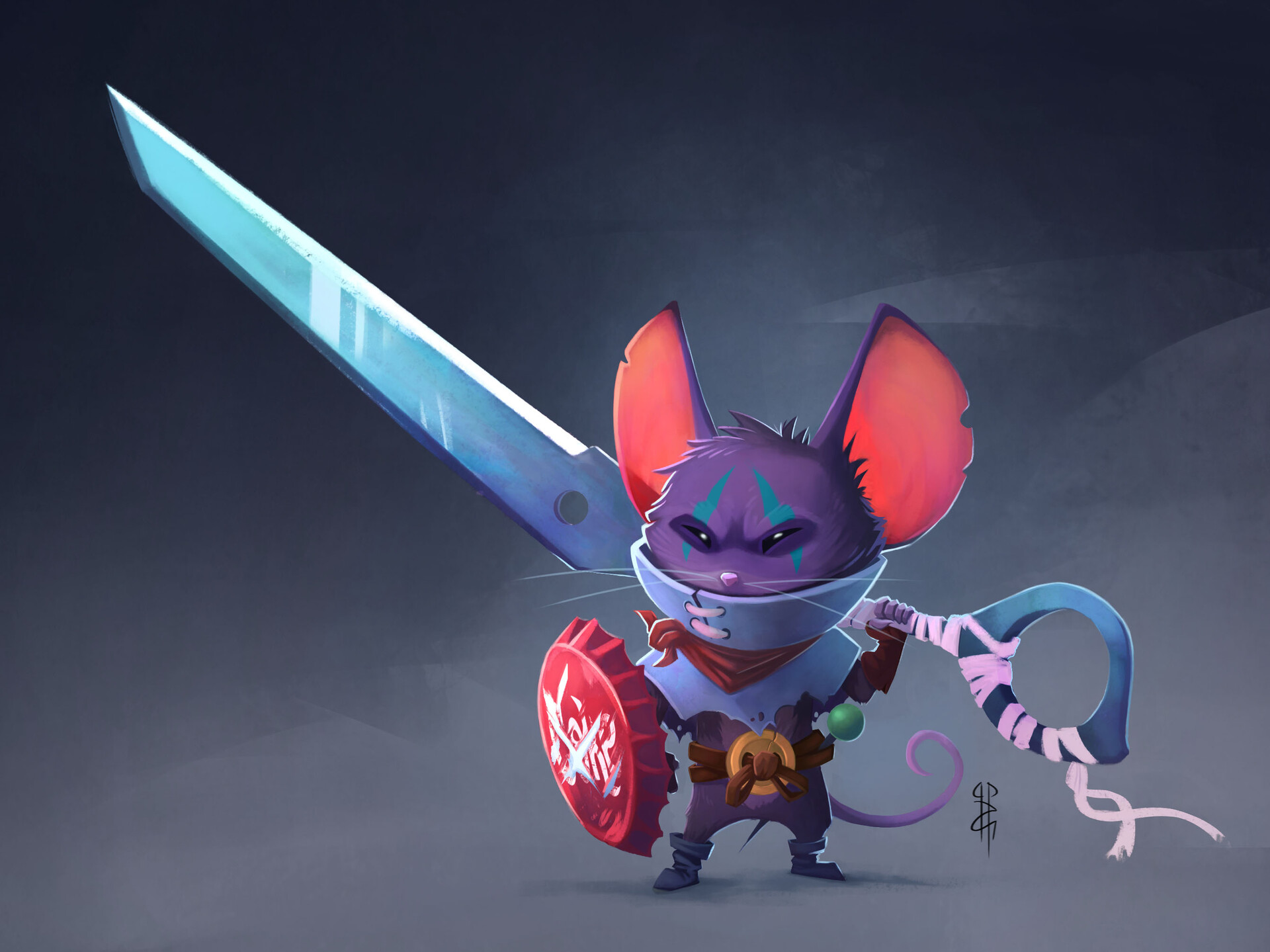This digital drawing showcases a character that could belong to a video game, manga, or fantasy book, set against a dark background. The focal point is a small, purple mouse positioned slightly to the right of center, standing out as the most colorful element in the otherwise gray scene. The mouse has a distinct ninja-like appearance, with a red shield fashioned from a bottle cap and a weapon made from one half of a scissor—wrapped in light purple or pink tape—that serves as a makeshift sword. The mouse dons a purple outfit, complete with a purple curly tail and a scarf, or bandana, around its neck. Its face is purple with reddish ears, aqua areas around its eyes, and something sewn over its mouth, adding to its detailed features. Enhancing its warrior-like aesthetic, the mouse is equipped with shoulder armor and a belt. The artist's signature is subtly placed slightly to the right of the mouse.